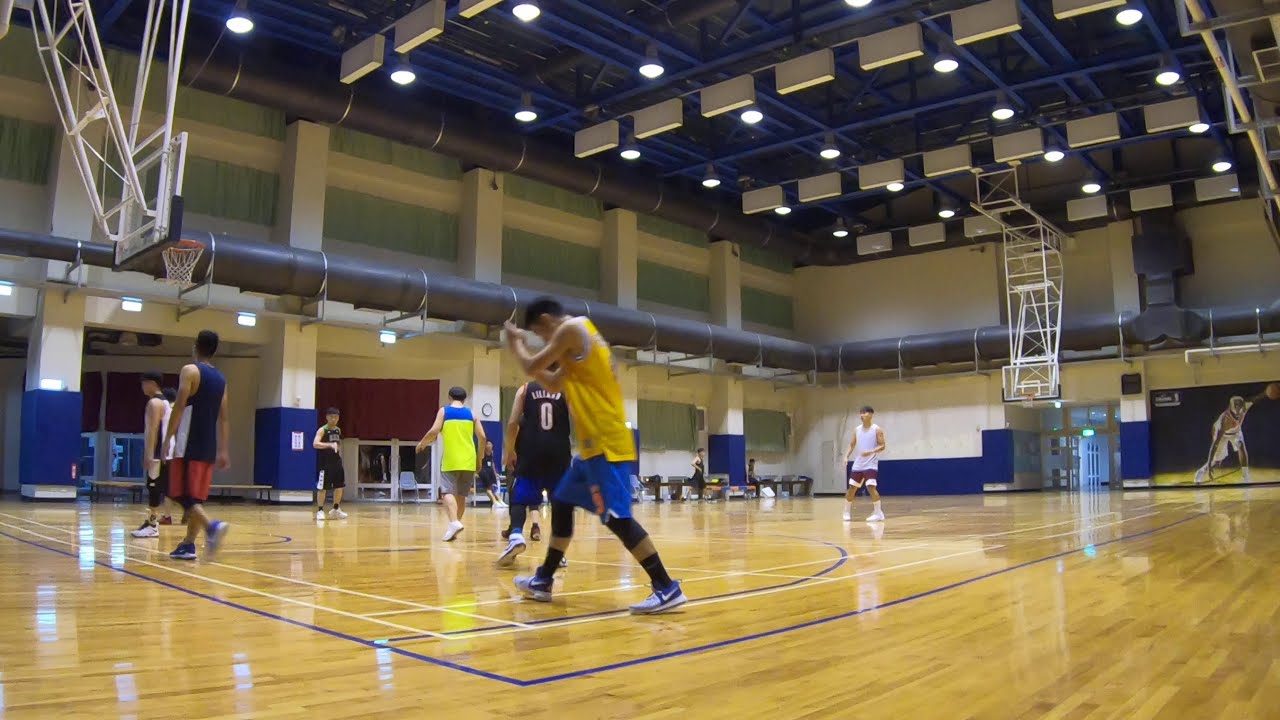The photograph captures a lively scene inside a brightly lit gymnasium, where several athletes are engaged in a basketball game. The gymnasium features high, dark blue ceilings with blue pipes and extensive ductwork along the walls. The court itself is distinctive with a shiny, wood-paneled floor highlighted by bright blue and yellow markings. In the center of the image, a number of players can be seen wearing various basketball uniforms. Closest to the camera is a player in a yellow top and blue shorts. Just behind them, slightly to the left, stands a player wearing a black top with the number zero and blue shorts. To their left is another athlete in yellow, followed by someone in black. Further to the left is a player donning a blue and red outfit, and next to them is another player in black and white. On the far right of the yellow and blue player is an athlete in a white and black uniform. Additionally, a poster depicting a basketball player in a crouched position can be seen on the wall to the far right, near some doors. The gymnasium appears to be a practice venue, as it lacks substantial spectator seating or bleachers. The bright lighting and bustling activity emphasize the energetic atmosphere of the game in progress.